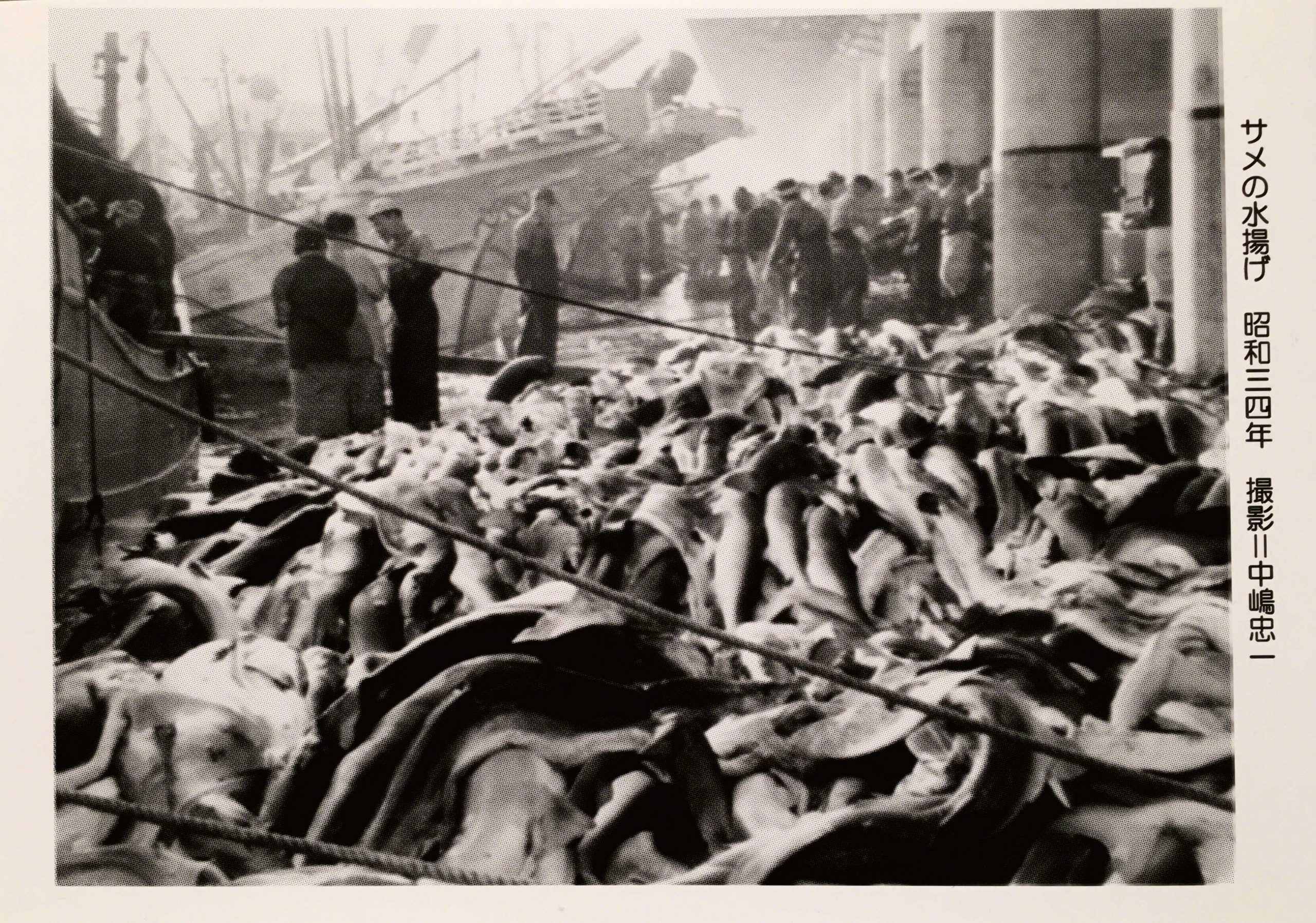The black and white photograph, framed by a light gray border on the bottom left and right, portrays a bustling dock area, possibly a fish market or yard. This gritty, old image, reminiscent of a vintage magazine or newspaper, captures the scene in remarkable detail. Central to the photograph are piles of fish being meticulously pulled in past multiple support pillars by several workers, some of whom are engaged in conversation. On the left of the frame, fishing vessels are seen unloading their hefty catches onto the dock, their bows jutting over the platform. The right side of the border features vertical black text in Japanese, adding an authentic touch to this historical snapshot.